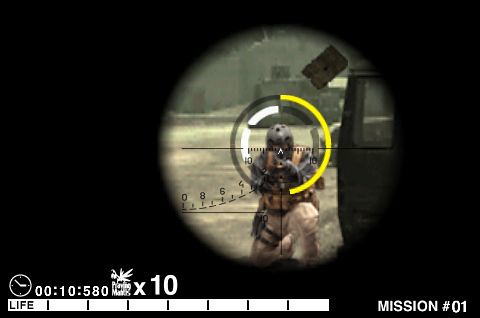This detailed screenshot from a first-person shooting video game features a sniper's perspective aimed at a soldier in a battlefield environment. The central focus is through the circular view of a sniper scope, equipped with a reticle centered precisely on the head of an army-clad soldier wearing a tan vest, tan pants, and a black helmet. The scope also displays viewfinder markings and numeric indicators for range and accuracy. The surrounding battlefield is characterized by gray stone pavement, smoky ambience, and a black truck, hinting at an intense military setting. At the bottom of the screen, a life bar and time indicator are visible, along with the text "MISSION 01" prominently displayed, indicating the current game mission.